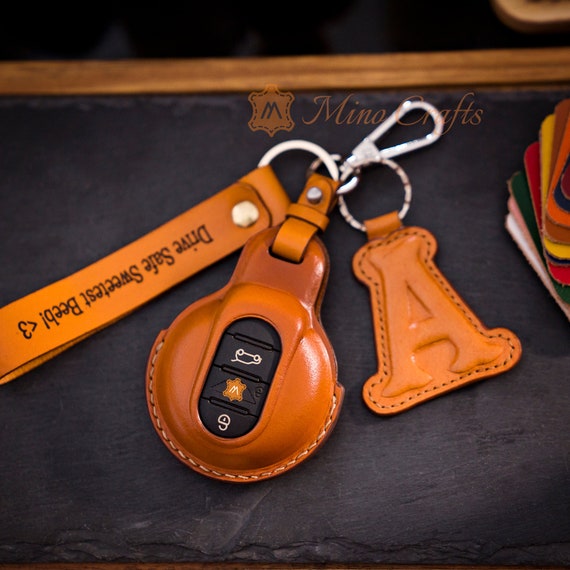This image showcases a meticulously crafted keychain set, likely advertised by Mina Crafts, set against a black background that resembles a chalkboard. Prominently made from medium orange leather, the keychain includes a wrist strap adorned with the words "Drive Safe Sweetest Bebe" and a heart symbol in brass. The key fob, secured within an oval-stitched leather holder, features buttons for unlocking doors and opening the trunk. Attached to the keychain is a silver ring with an embossed leather letter "A" and an orange circular holder with a black 'W' button, enhancing its versatility. To the right, a stack of differently colored leather swatches suggests customizable options for the leather accessories.